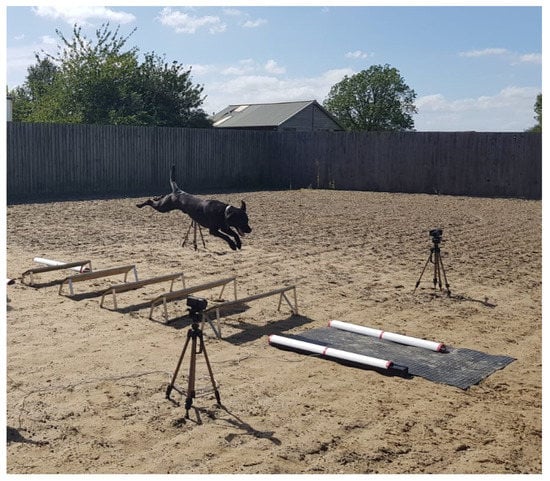In this color photograph, taken outdoors during the day at a dog training facility, a black dog is captured mid-air as it jumps over a series of wooden hurdles set up in a large, entirely dirt-covered, fenced-in area. The fence is dark gray, and beyond it, the tops of two trees and the gray roof of a building are visible beneath a light blue sky dotted with white clouds. The hurdles are spaced apart, and the dog appears to be aiming for a black landing pad with white barriers on either side. Positioned to capture this moment, two video cameras on tripods flank the landing pad. The area is devoid of any other animals or people, focusing entirely on the dog's impressive leap.